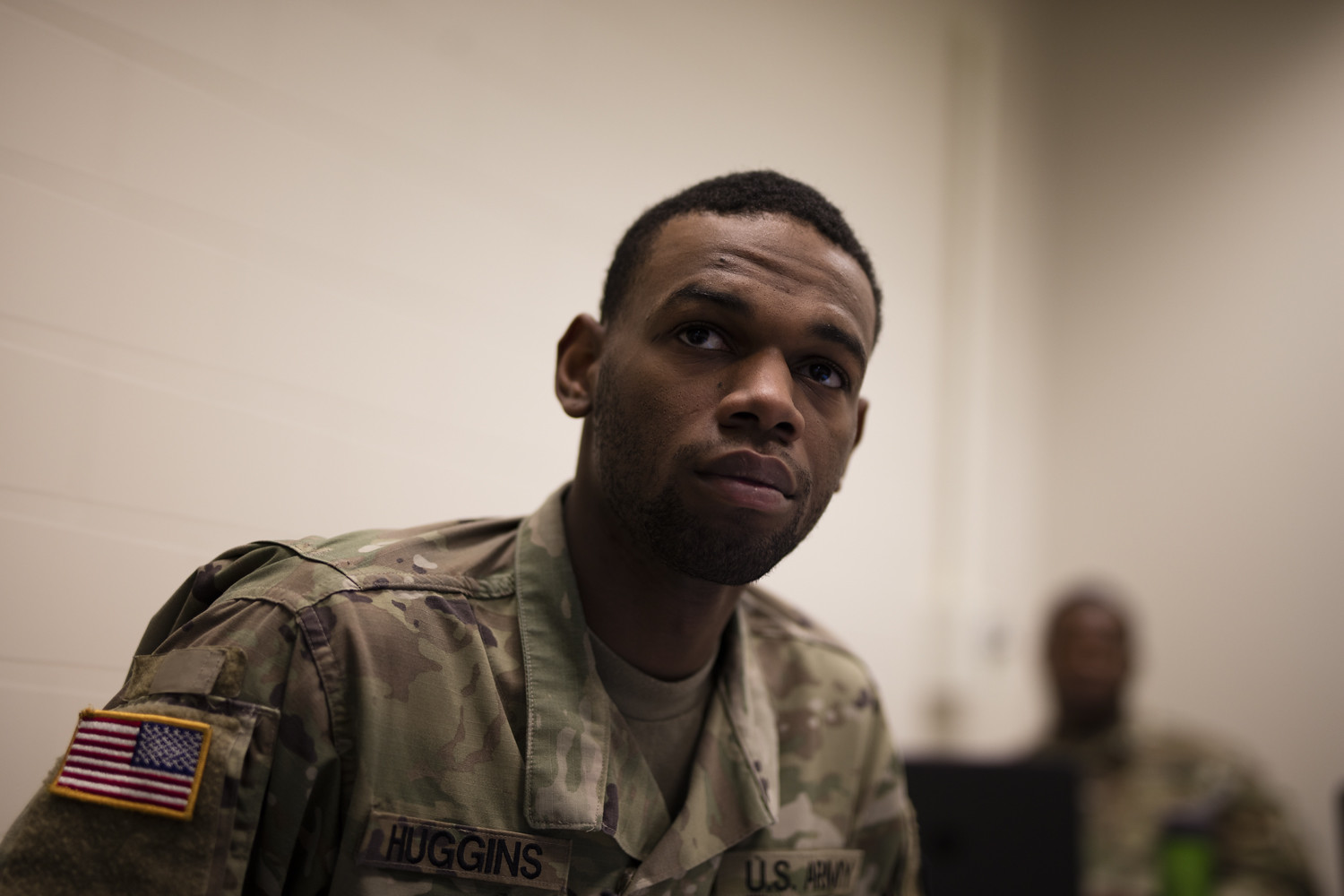This image portrays a close-up, side-profile portrait of an army soldier named Huggins, identifiable by his embroidered name tag on the left side of his camouflaged uniform. The uniform design consists of the typical green and brown pattern associated with the U.S. Army, and also features a U.S. Army tag on the right side of his chest. Prominently displayed on his left shoulder is a patch of the U.S. flag with a yellow border. The setting appears to be inside a room with white walls. In the blurred background, another soldier can be seen working on a laptop, though this secondary figure is significantly out of focus, emphasizing Huggins as the central subject of the image.